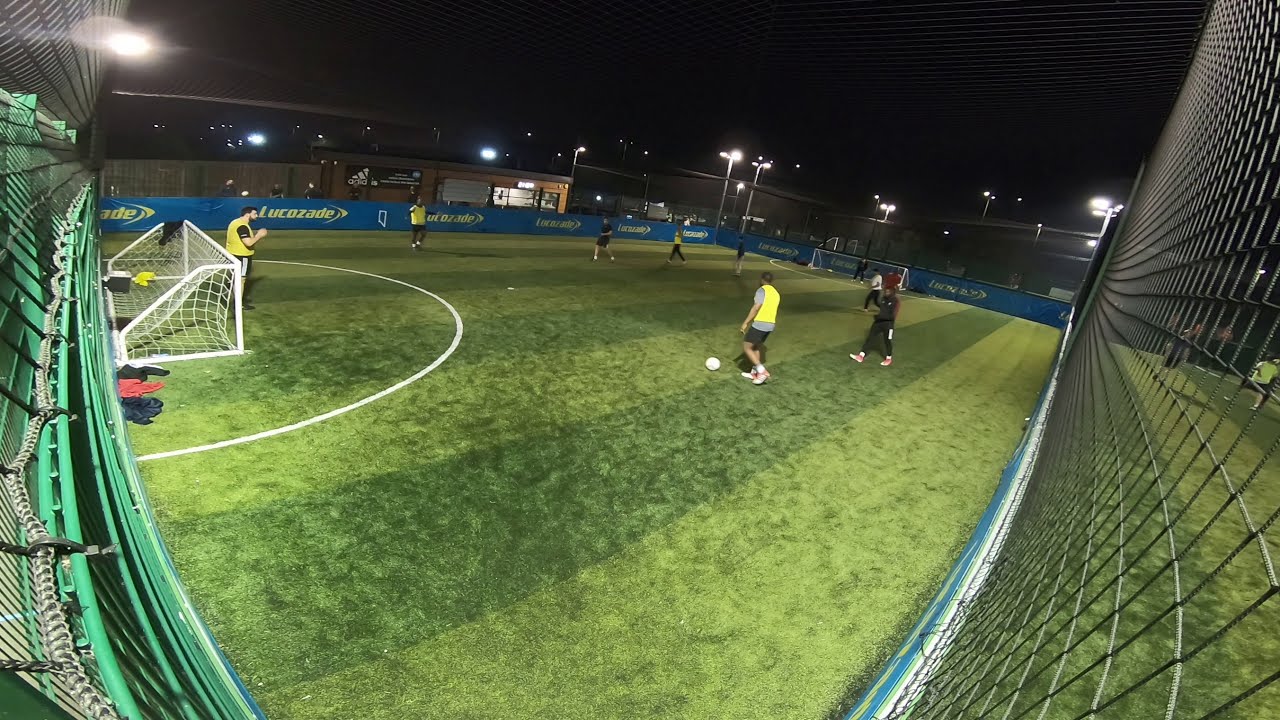In the photo, a meticulously mowed green grass soccer field is illuminated under a dark nighttime sky. The field, bordered by surrounding lights, features alternating light and dark green mowing lines. A blue awning with yellow text reading "Lucozade" encircles the base of the field. The scene, which appears to be a practice session due to the sparse presence of spectators, includes several players visible across the field, most prominently a player in a yellow shirt near the center-right, preparing to kick a soccer ball positioned on the grass. Nearby, another player in a darker uniform and possibly a referee can be seen. To the left, the goalpost is visible, framed by the fencing that runs along both the left and right sides of the image. The setting is calm and focused, with the primary colors being green, yellow, blue, and black.